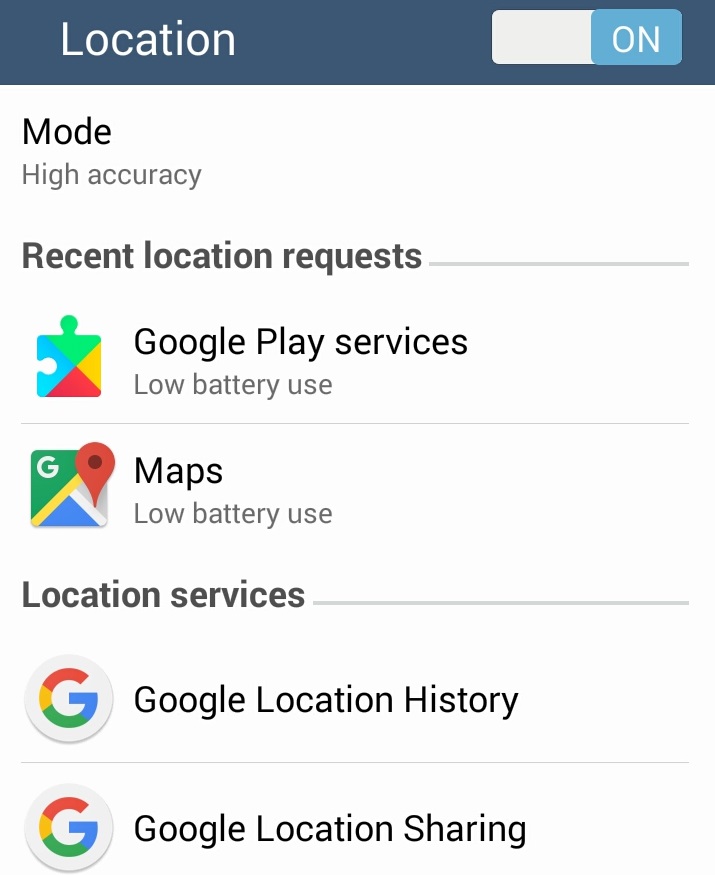The screenshot depicts the location settings interface on a smartphone. The top inch of the screen features a dark blue header. On the left side of this header, large white letters display the word "Location." On the right side, there is a toggle switch. The left part of this switch is white and the right part is light blue, with the word "On" written in white.

Beneath the header, the background turns white. In the top-left corner, bolded black text reads "Mode," followed by the label "High accuracy" in a slightly off-black, grayish color. Below this section, there is a small space before the bolded black heading "Recent location request" appears. This heading is underlined by a gray line extending to the right side of the screen.

Under the heading, the first item listed has a multi-colored puzzle piece icon, with green on top, yellow on the right, red on the bottom, and blue on the left. To the right of this icon, bold black text reads "Google Play Services," and below it is the description "Low battery use" in an off-grayish black font. A line separates this item from the next.

The subsequent item shows the Google Maps icon, accompanied by the text "Maps" in black. The description "Low battery use" follows in a similar off-grayish black font.

Further down is another bolded black heading, "Location services," underlined by a gray line extending to the right. Below this line, a circular icon with the Google 'G' precedes the text "Google Location History" in black. Another thin gray line is present, followed by another Google 'G' icon and the label "Google Location Sharing" in black text.